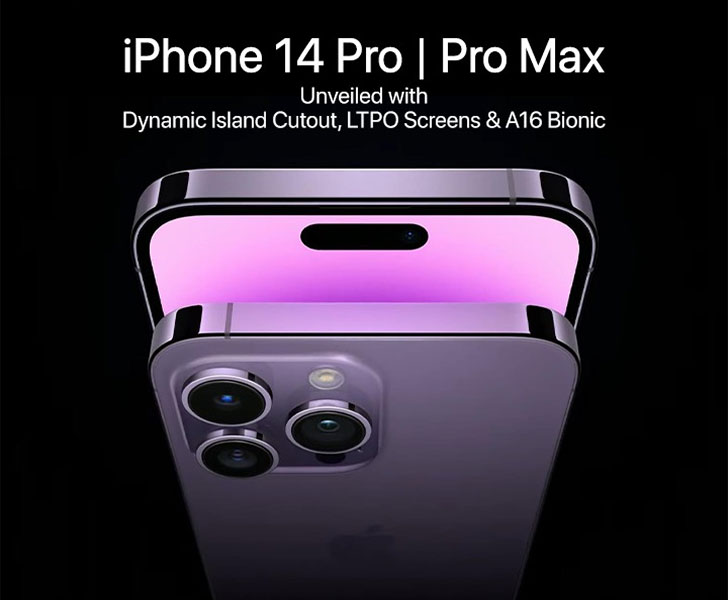In this captivating image, set against a stark black background, bold white text prominently announces the "iPhone 14 Pro." A sleek white line divides the text, below which "Pro Max" is unveiled, highlighting features such as the Dynamic Island cutout, LTPO screens, and the powerful A16 Bionic chip. The centerpiece of the image is an exquisite light orchid-colored iPhone 14 Pro. The phone is artistically doubled, with the top portion slightly pulled down to reveal a portion of the screen. The screen transitions from a dark purple at the bottom to lighter shades of purple towards the top, accented by a distinctive black oval shape at the upper center, indicating the new Dynamic Island cutout. The phone’s back showcases three elegantly designed camera lenses in silver and black, along with a small white circle, possibly denoting an additional sensor. All of this is framed within a large box that mirrors the phone’s elegant orchid hue.